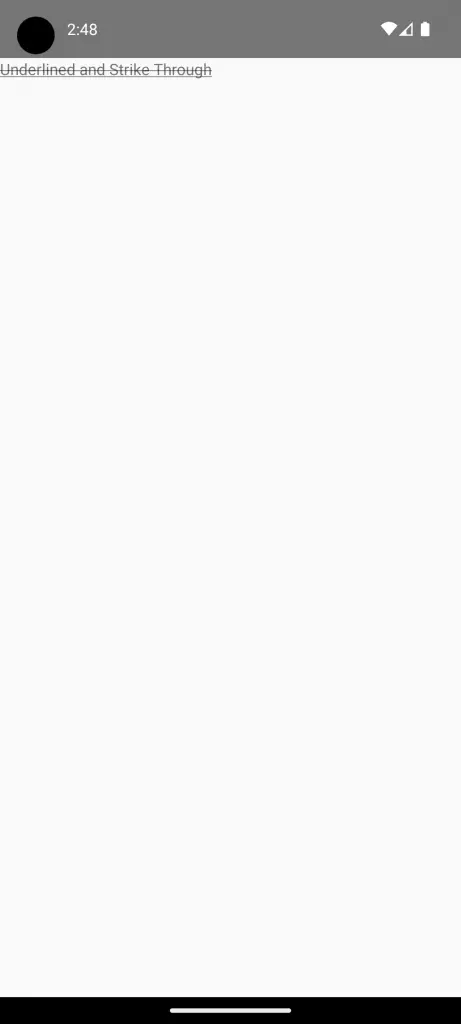The image features a top section with a gray border that contains a black oval with the digital time display of 2:48. Adjacent to the time display are icons indicating Wi-Fi connectivity with two out of four bars, and a battery icon with an indeterminate charge level. Below this section, the background shifts to light gray. On the top left corner of this light gray area, there is dark gray text which is underlined and reads "underline and strikethrough." The central portion of the image is predominantly empty space, creating a minimalist aesthetic. At the very bottom, there is a black strip stretching the full width of the image, adorned with a thin white line running horizontally through its middle. The overall feel of the image is sparse and clean, with focus on the simple interface elements and ample blank space.